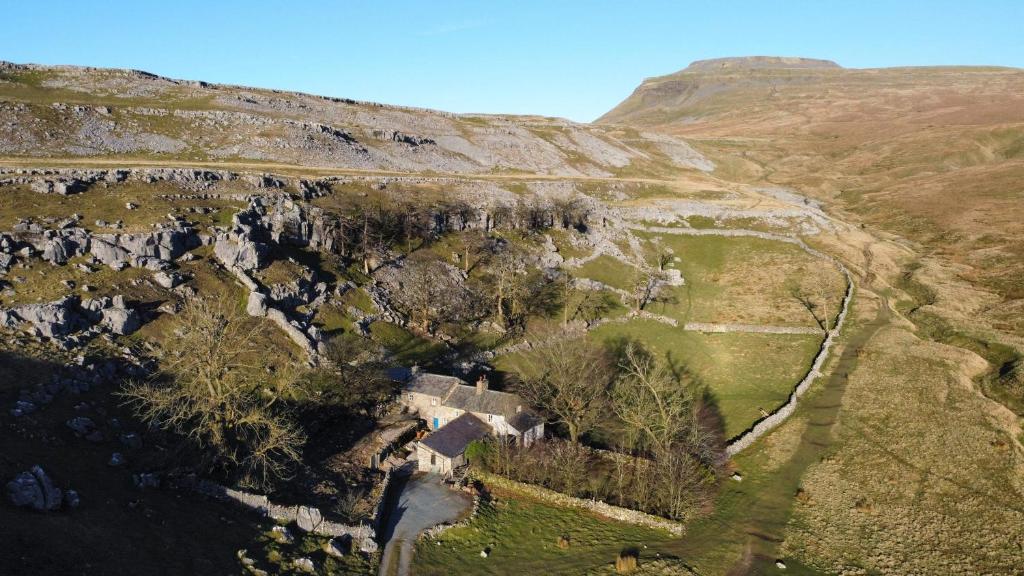An aerial view reveals a picturesque rural scene nestled in a mountainous valley. At the center of the image is a three-section stone house with a blue door and a grey roof, distinguished by two brown chimneys. The tallest portion of the house is on the left, the shortest on the right, and a smaller section at the front. Surrounding the house is a stone wall that curves and connects to another rock wall, enclosing the backyard and adding to the rustic charm. The area is dotted with dark gray rocks, patches of dehydrated green grass, and clumps of trees, all contributing to the isolated and serene atmosphere.

The surrounding hills and mountains exhibit a palette of greenish-brown and dark green hues, with lighter brown colors adorning their sides. The sky above is a bright, clear turquoise blue, free of clouds, suggesting fair weather. On one side of the mountains, a road is visible. To the top left of the image, there is mostly bare rock interspersed with patches of greenery, while a small canyon can be seen in the upper right. It's late in the evening, evident from the long shadows cast across the landscape, enhancing the tranquility and remoteness of this rural haven.